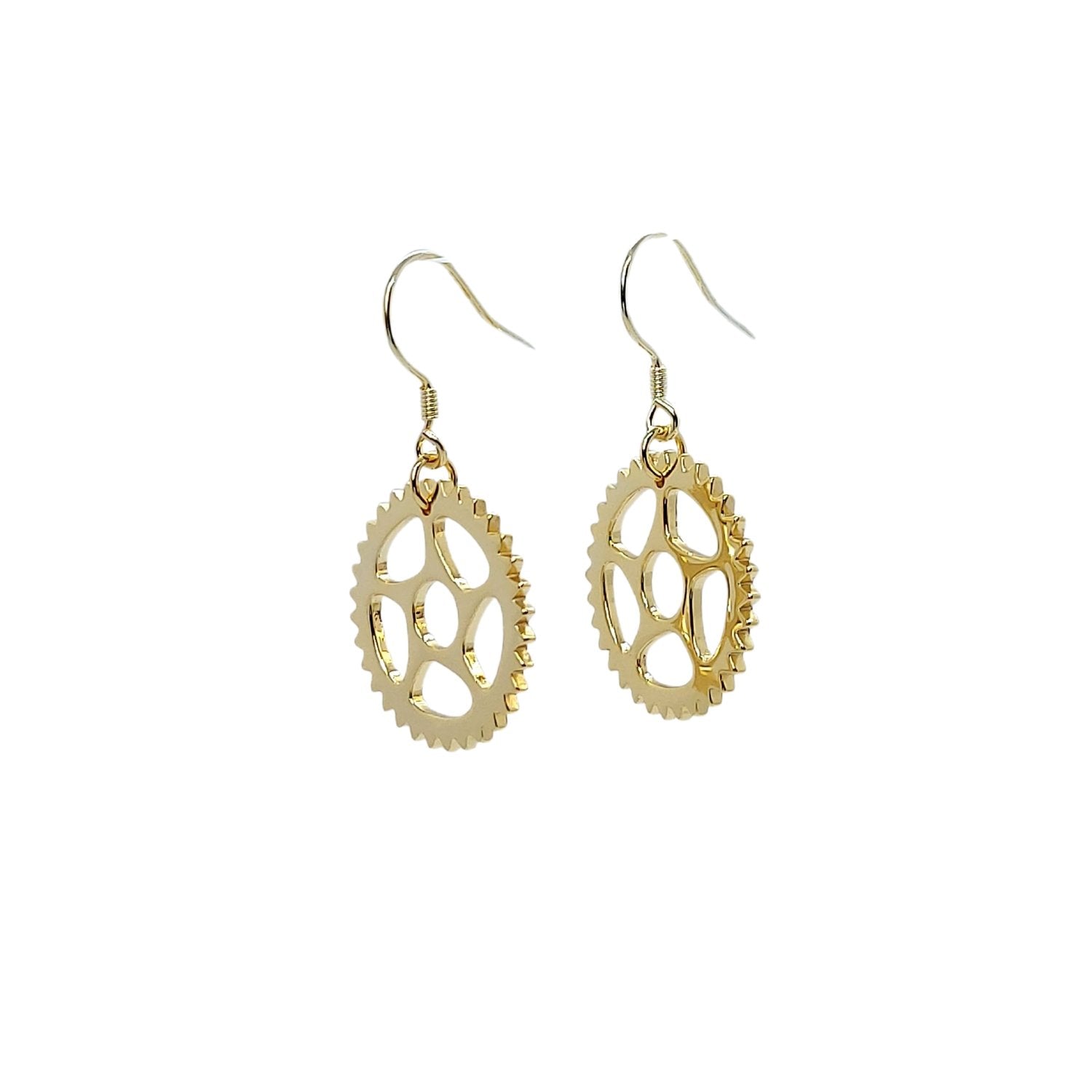This image is a studio photograph on a completely white background, showcasing a pair of gold-plated earrings designed to resemble gears. The earrings feature hooks with sharp tips and multiple coils leading to a noose-like end that attaches to the gear-shaped pendants. Each gear has five spokes converging at a central circular hub, surrounded by numerous small, pointed teeth along the outer edge. The surface of the gears is highly polished, giving them a shiny, reflective appearance. The design includes intricate, cut-out patterns within the gears to reduce weight, possibly invoking the aesthetic of machinery or old watch components. The absence of any objects for scale makes it difficult to determine the exact size, though they appear to be roughly the diameter of a dime.